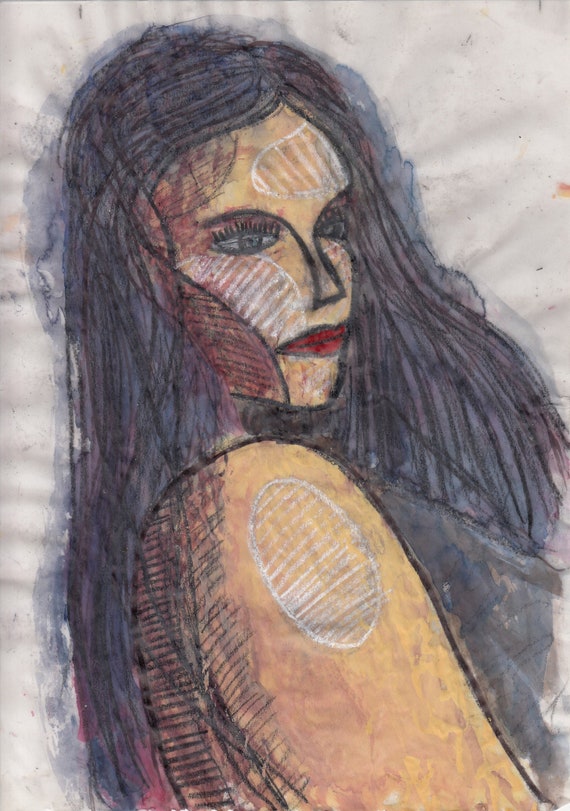The image is a detailed artist's drawing of a beautiful woman, executed with pencils and watercolor on a textured white background. The woman, positioned with her back partially toward the viewer, appears to be gazing to the right. She has long, flowing dark hair with subtle blue and purple highlights. Her hair is parted slightly to the side and features distinct black lines around the edges with a smeared or water design effect.

Her strong facial features include bright blue eyes with long eyelashes, a slender, well-defined nose highlighted with thick black lining, and full red lips. Her face and right cheek are adorned with white circles and intricate white line patterns, which also appear on her upper right arm within an oval shape, creating a consistent design element across her skin.

She is wearing a sleeveless top, which seems to alternate between dark, possibly black, and hints of blue and pink hues. The background is predominantly grayish-white with darker ink accents. Overall, the composition is both striking and intricate, combining sharp, defined lines with delicate watercolor shading.